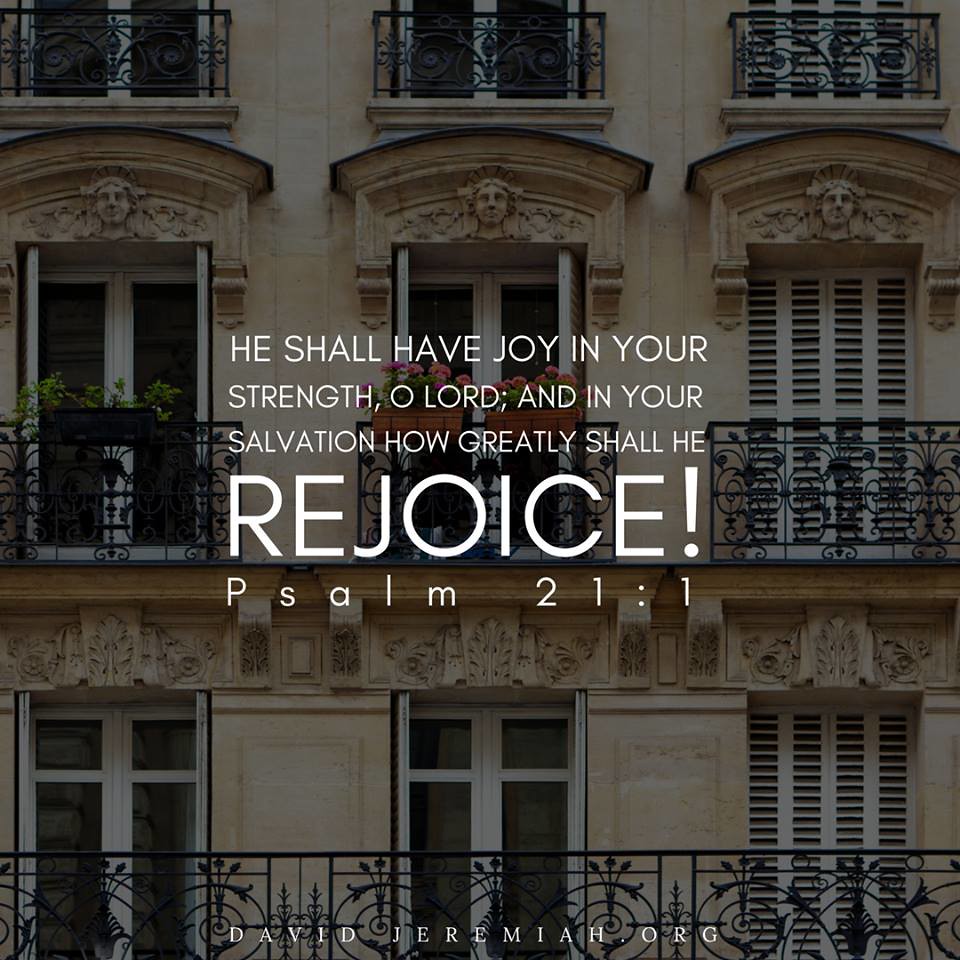The image features an imposing stone building, reminiscent of European architecture, possibly an old hotel or a grand apartment complex, bathed in a subdued lighting that makes the scene appear somewhat faded. The structure showcases nine elegant, full-length windows, each adorned with distinct wrought iron railings featuring intricate designs. Above each window, there is a finely chiseled stone carving of a man's face situated within an arched frame. Superimposed over this striking architectural backdrop is a Bible verse from Psalm 21:1, written in bold white sans-serif font: "He shall have joy in your strength, O Lord, and in your salvation, how greatly shall he rejoice." The word "rejoice" stands out prominently, emphasized with an exclamation point. At the bottom of the image, the web address DavidJeremiah.org is subtly printed in small white letters, tying the inspiring message to its source.